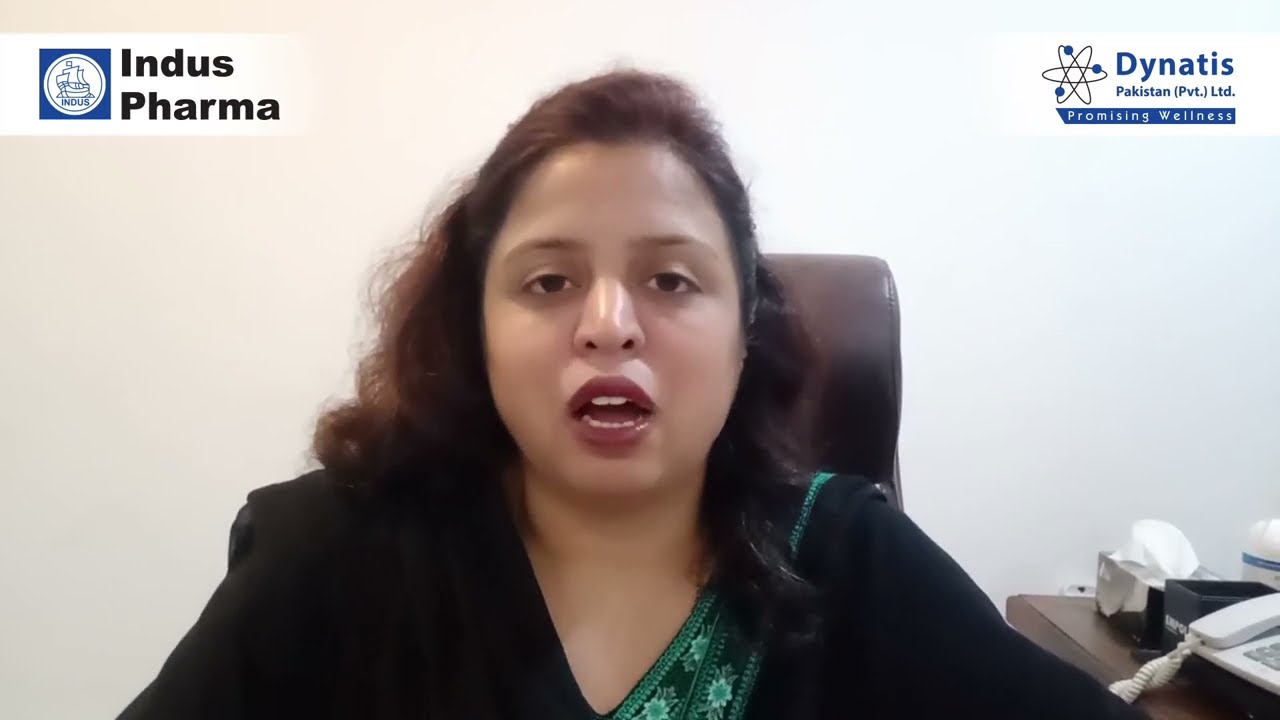The image depicts a woman of darker complexion, likely Indian, who appears to be mid-sentence during a video call. She has wavy, brown hair cascading below her shoulders, brown eyes, and is wearing dark red lipstick. She is dressed in a black blouse with green floral trimmings. The background is a light, whitish wall, suggesting an indoor office setting. The top left corner features a logo in a blue square with a round white circle inside, containing the image of a large boat with several sails and the text "Indus Pharma" in black. The top right corner bears the logo "Dynatis Pakistan LTD Promising Wellness." To the right of her, part of a desk is visible with a white telephone and a tissue box. Her office chair is also partially visible.